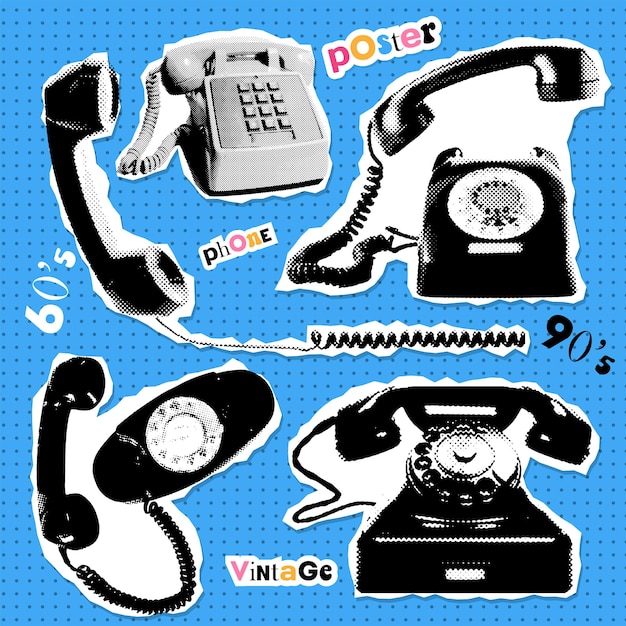This large, square, computer-generated image features a vibrant design resembling a collage of sticker-like elements against a blue polka dot background composed of very small, slightly darker blue dots. The artwork showcases a variety of black-and-white cutout telephones from different eras, predominantly featuring rotary dial phones.

In the upper left corner, there’s a vintage phone handle with its cord stretching across the center, accompanied by the word “90s” noted beside it. Just to the right, another phone appears with its circular dial visible, positioned on its receiver, and the word "POSTER" spelled in colorful, cutout-style letters next to it.

The upper right corner presents another rotary dial phone, black in color, with the handset noticeable just above it. Moving to the lower left, an oval-shaped phone is displayed, next to the word “VINTAGE.” Finally, the lower right section features another black rotary dial phone, completing the diverse assembly of analog communication devices.

The entire composition has a refined, risograph feel, with the juxtaposition of monochromatic phone illustrations and colorful text elements creating a visually engaging homage to telephones from the 60s to the 90s.